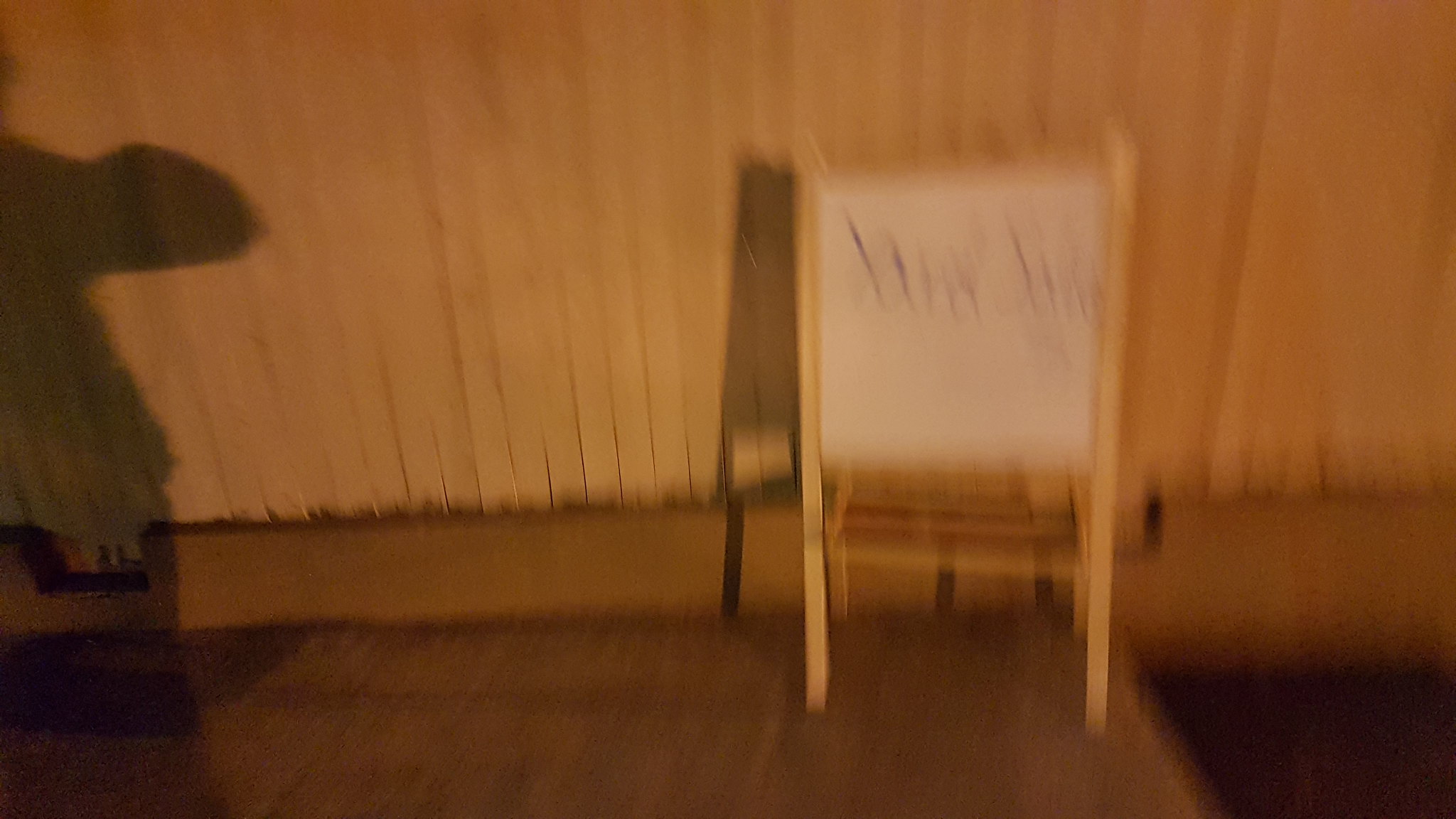The blurry photograph captures a scene that is approximately 50% wider than it is tall. Dominating the center is a child's standing easel made of light-colored wood. Attached to the easel is a large whiteboard where some illegible text, written in black or green marker, occupies the upper portion. The background features a slatted wooden wall or fence composed of vertical boards, presented in a light color, transitioning to a medium brown baseboard and floor, possibly made of wood, though one perspective suggests it might be concrete with patches of grass around it. There is a notable shadow cast on the right side, hinting at the presence of a light source behind the camera, and potentially a silhouette resembling a person. Additionally, a darker brown color runs along the bottom of the fence, which might signify some debris. The easel appears slightly tilted to the left, and there is a rung between its legs casting a shadow on the ground.